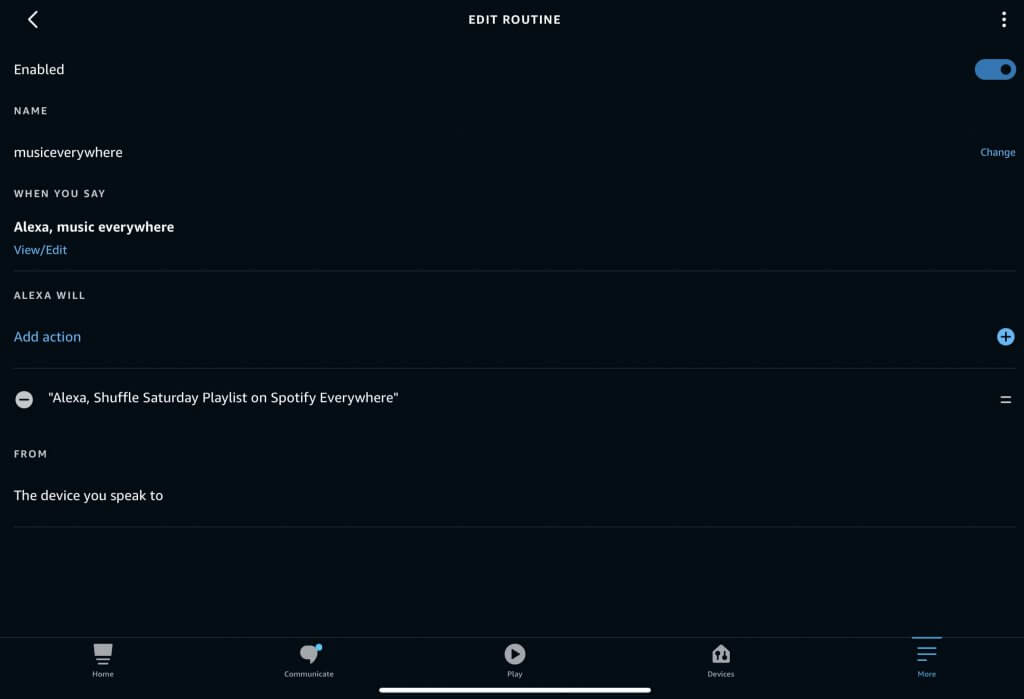The image displays a section of a website with a predominantly black background. At the top center, in bold white capital letters, the text "EDIT ROUTINE" is prominently displayed. To the right of this title, there is a vertical ellipsis (three dots aligned vertically), indicating additional settings or options. On the left side, there is an arrow key pointing either left or right, allowing navigation.

Beneath the title, a menu option labeled "Enabled" appears, with a sliding toggle button on the far right. This button is switched on, revealing a blue background.

Further down the interface, on the left, the text "Name" is followed by the phrase "Music Everywhere." Below this, the text reads, "When You Say, Alexa, Music Everywhere," with a clickable "View/Edit" link in blue text following. The instructions then state, "Alexa will add action."

On the right side, next to these instructions, a blue circle featuring a white plus sign (+) suggests the addition of new actions or commands.

Continuing down the left side, there is a white circle with a minus sign (-) inside, corresponding to an existing action: "Alexa, Shuffle Saturday Playlist on Spotify Everywhere." To the right of this action, an equal sign (=) is displayed, likely indicating configurable options.

At the bottom of the segment, the text "From the Device You Speak To" is shown, clarifying the source of the commands.